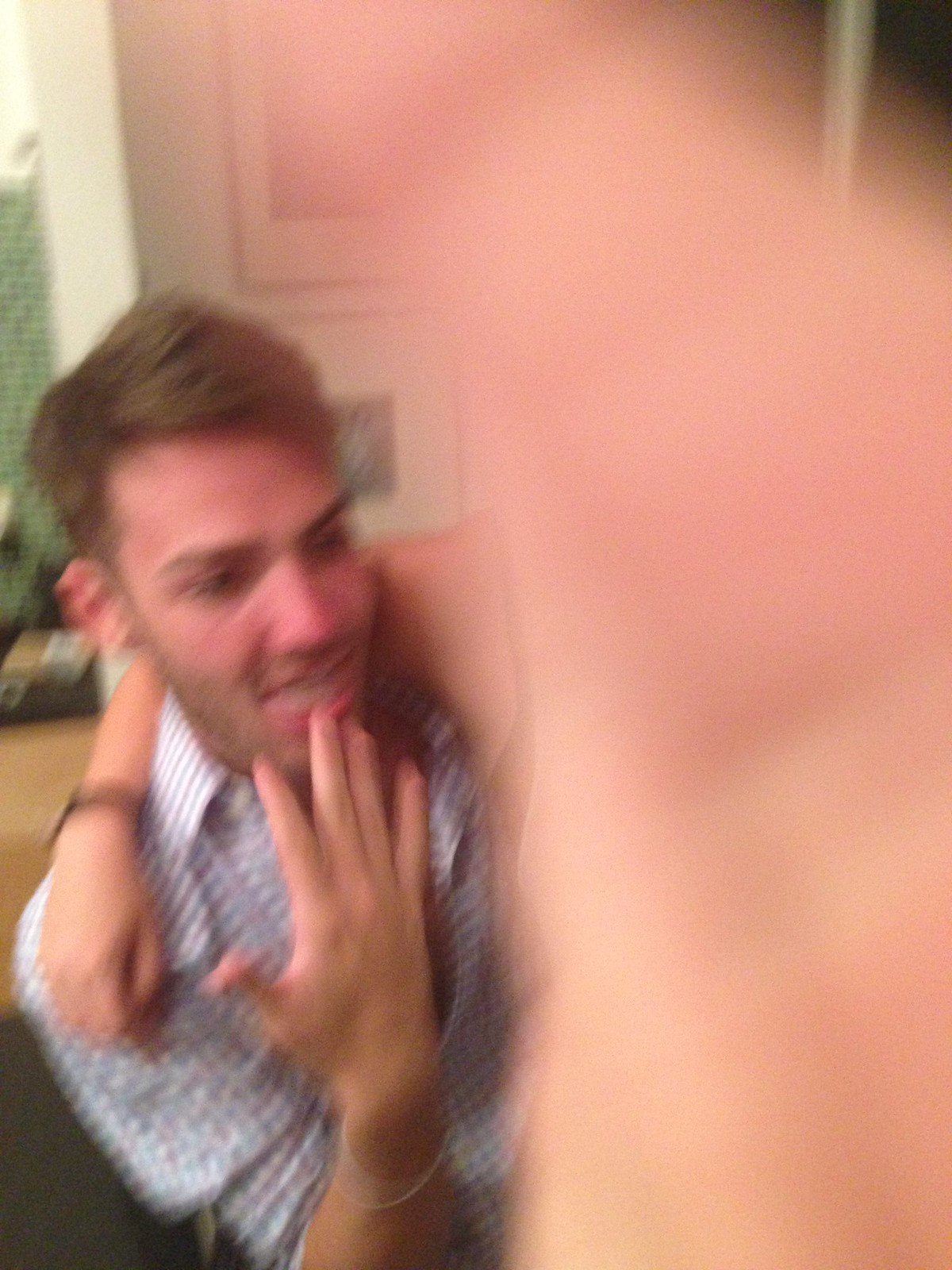This photograph captures a playful and chaotic moment between two people. Dominating the right side of the image is a blurry hand, partially obstructing the scene. Behind the hand, we discern a Caucasian man with light brown, fluffy hair and a five o'clock shadow, possibly indicating a slight intoxication suggested by his pink blush. He stands in front of a cream-colored wall adorned with various framed pictures. The man, dressed in a blue and white checkered shirt with sleeves rolled up to his elbows, is making a silly face, finger in his mouth and eyes cast downward, not looking at the camera. Another person's arm, clad in a tank top, is draped around his neck, contributing to the image's obscurity. The exact intention—whether accidental blurriness or deliberate anonymity—remains unclear, but the photograph vividly documents a lighthearted, spontaneous interaction.